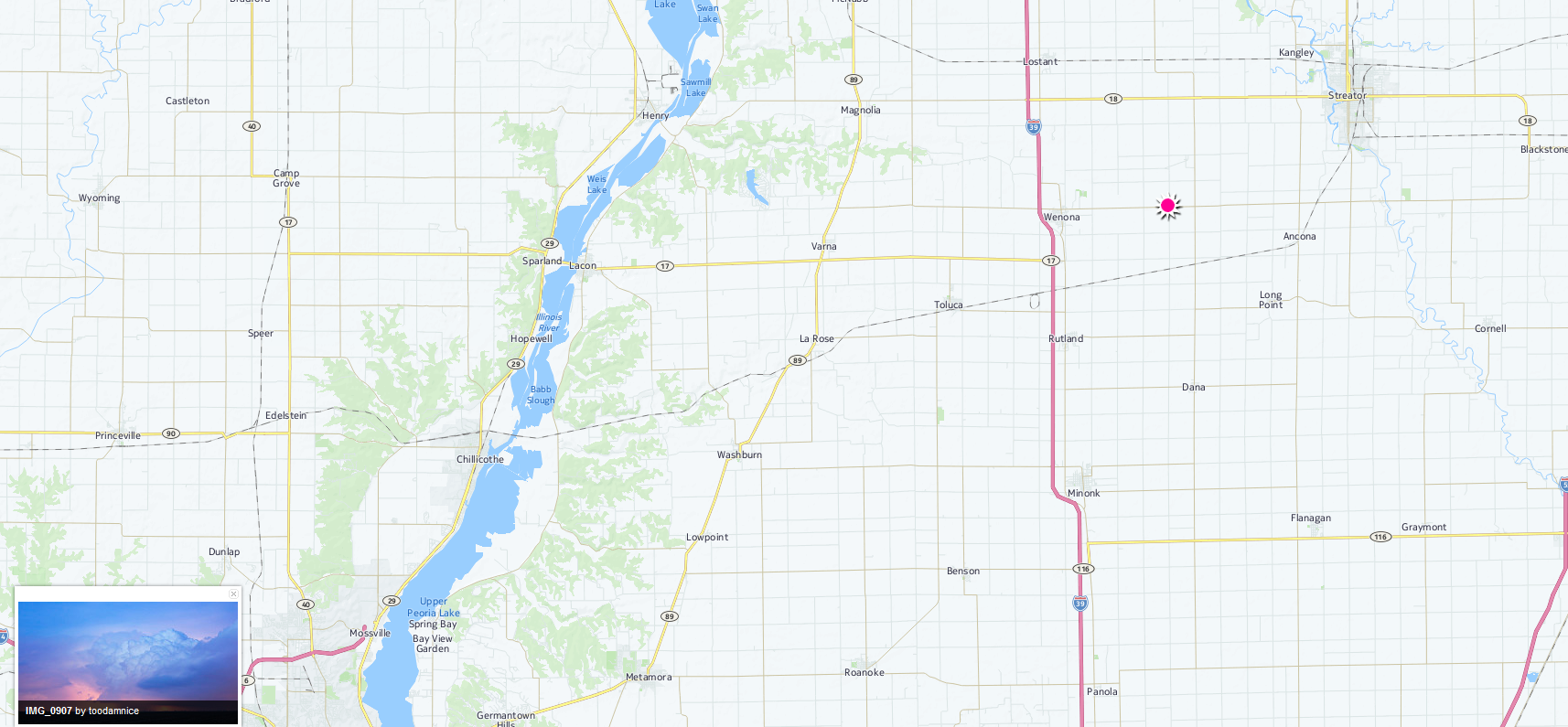This image depicts a detailed map featuring various roads and natural landmarks. In the bottom left-hand corner, there is a small inset rectangle. At the top of this rectangle is a white line, and at the bottom, there is a black line containing unreadable text. Between these lines is an image displaying a blue sky with clouds and a hint of a pink sun. The map itself is crisscrossed with roads marked in different colors; pink lines indicate interstates, yellow lines signify major roads, and slightly different shades of yellow represent smaller roads.

On the left-hand side of the map, a prominent river runs vertically from the bottom to the top, bordered by green splotches indicating forested or grassy areas. On the right-hand side of the map, a smaller stream or brook, depicted as a blue squiggly line, meanders across the landscape. The map is further divided into grids or squares, each containing an intricate network of intersecting roads.